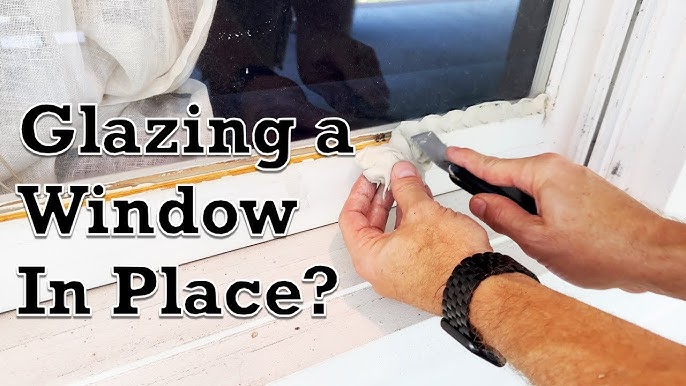The image is a close-up from a DIY tutorial likely introducing a video on glazing windows. Dominating the left side of the image, black text reads, "glazing a window in place?" The focal point features a person actively glazing a white, weathered wooden window. The individual, wearing a black Apple watch on their left wrist, uses a spatula to apply a gray-white putty along the windowpane. Their right hand grasps a tool that resembles a razor with a black handle. The scene shows the glass window with pushed-aside gauzy curtains, suggesting darkness outside. The composition captures the intricate details of the process, highlighting both the act of glazing and the well-worn texture of the window and sill.